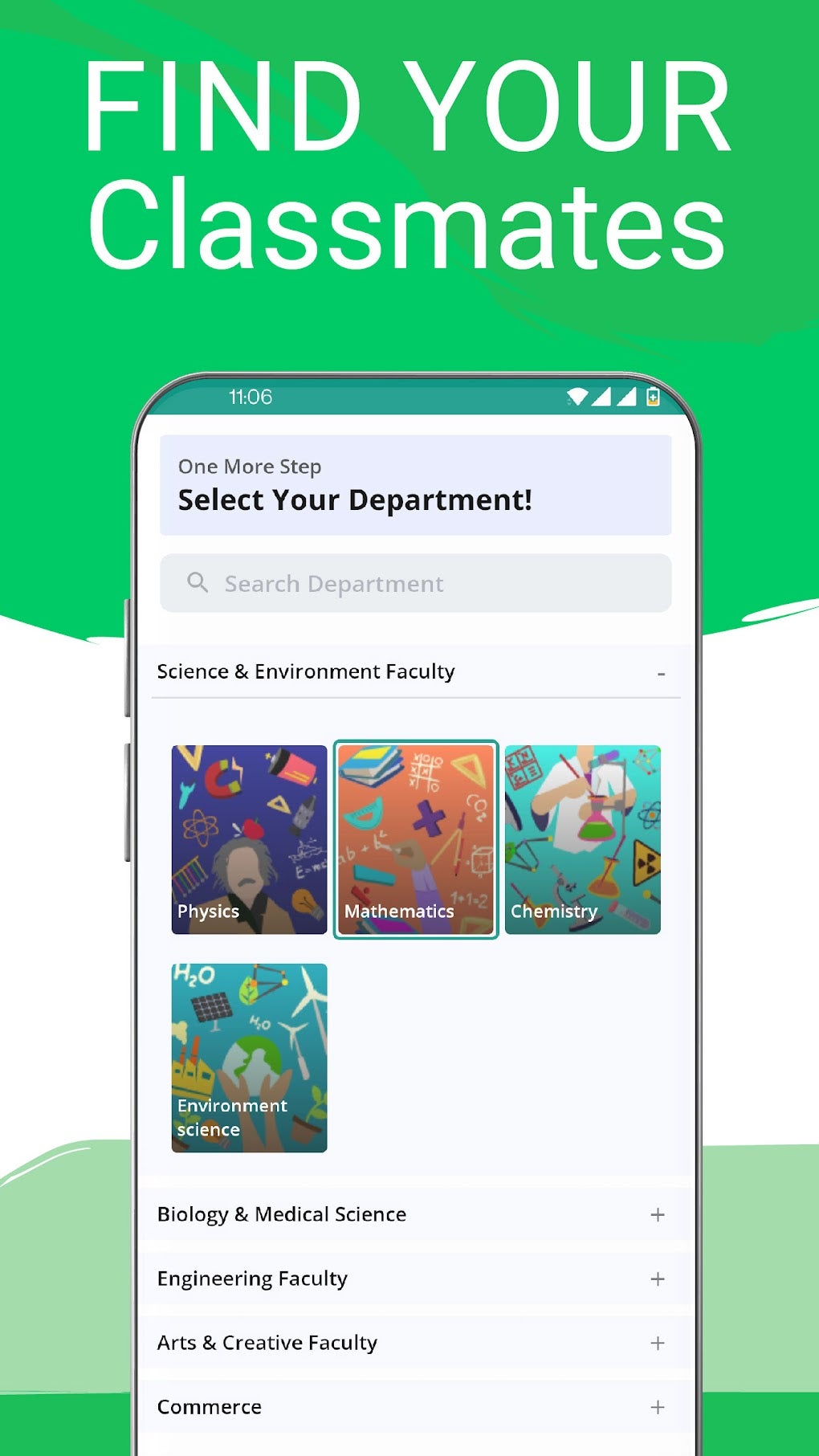The image appears to be an advertisement for a webpage designed to help users find their former classmates. At the top of the ad, a green banner with white lettering reads "FIND YOUR" in all caps, and just below it, "Classmates" with a capital C. Below this header, there's a graphic of a smartphone displaying the text "One more step: Select your department."

The ad showcases different departments, each represented by a colorful section and an associated illustration. For example:

- **Physics**: Featured on a bluish background with various scientific icons floating in the air. A cartoon man is depicted next to it.
- **Mathematics**: Displayed with an orange background, showing various mathematical symbols. Arms appear to be holding something up.
- **Chemistry**: Illustrated with an image of beakers and lab equipment, accompanied by a person in a white lab coat. Only the body of the cartoon character is visible.
- **Science**: Depicted on a blue background with hands holding up a globe along with other scientific symbols.

Below these sections, additional departments are listed as clickable options:
- Biology & Medical Science
- Engineering Faculty
- Art & Creative Faculty
- Commerce

The overall background of the webpage is white, while the text is predominantly blue.